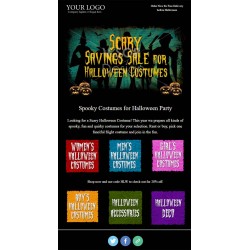A small, low-resolution screenshot appears to depict a Halloween-themed advertisement or social media post. The image quality is poor, making finer details difficult to discern. In the top left corner, the text "Your Logo" suggests a placeholder for a company's logo. At the bottom of the image, the footer includes circular social media icons for Twitter (also known as X), Facebook, and an unidentified green circle icon.

The main graphic features Halloween-themed elements, including pumpkins, and prominently displays the text "Scary Saving Sale for Halloween Customers" in bright yellow. Below this central text, there are six colorful square boxes that appear to serve as hyperlinks to different sections of a website. These boxes are labeled as follows:
- Women's Halloween Costumes
- Men's Halloween Costumes
- Girls' Halloween Costumes
- Boys' Halloween Costumes
- Halloween Accessories
- Halloween Decor

This image likely aims to guide users towards various Halloween-related products available on the advertiser's website.